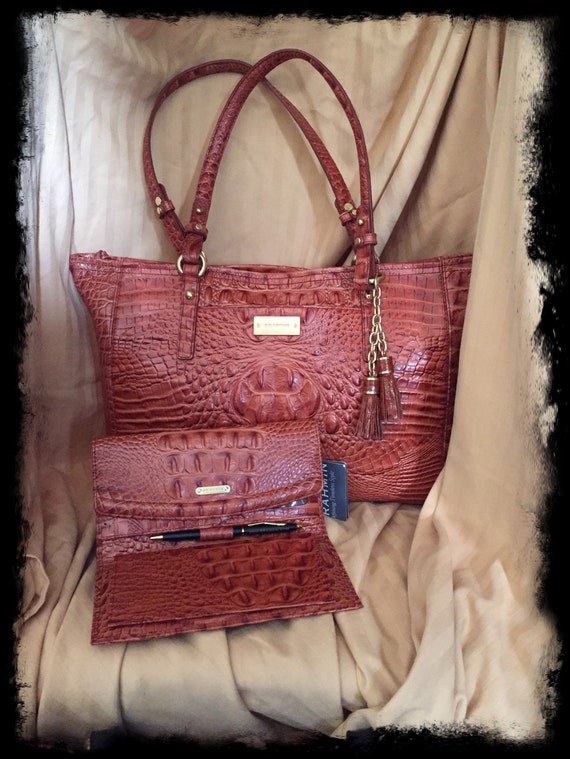The image showcases a luxurious display featuring a large handbag and a matching clutch wallet, set against an indoor backdrop of off-white beige wrinkled cloth. The centerpiece is a dark Sedona, Melbourne tote from the vintage Brahmin collection, crafted from crocodile-embossed Italian leather in a rich, burgundy rust-red hue. The tote, an exotic and expensive Australian piece, exhibits intricate leather detailing with droplets and lines, adding to its opulent look. It features two handles, a gold tag, and decorative tassels with a gold chain. In front of the tote, the matching clutch wallet is open, revealing a black pen inserted in its middle. The wallet, adorned with a little gold tag, complements the tote perfectly, completing the elegant display.